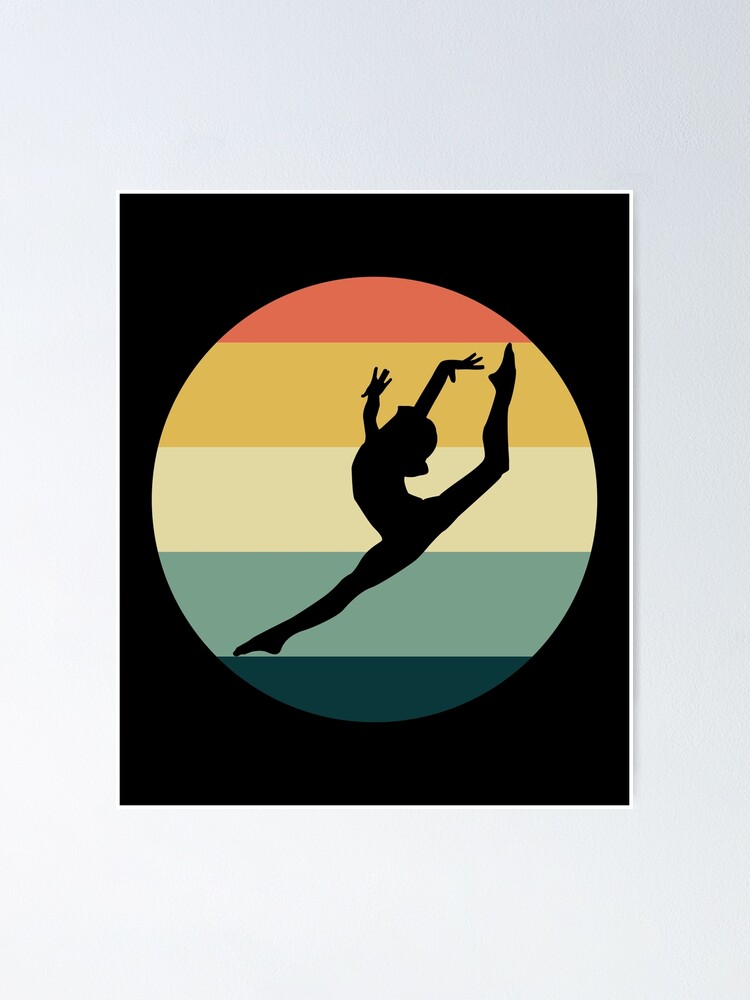This is a modern, illustrated poster featuring a striking silhouette of a ballet dancer in a dramatic side-view splits pose, standing on one foot with the other leg extended straight above her head. Her fingers are spread out, and her head is tilted back gracefully. The dancer is centered in a multi-colored circle composed of five horizontal layers, each with a distinct color: red at the top, transitioning to yellow, cream, teal, and finally a darker green at the bottom. This vibrant circle contrasts sharply against the surrounding black background, creating a compelling focal point. The entire composition is framed within a black square, standing out against the larger blue backdrop of the poster. This visually captivating artwork celebrates the elegance and strength of ballet through its bold use of color and striking silhouette.